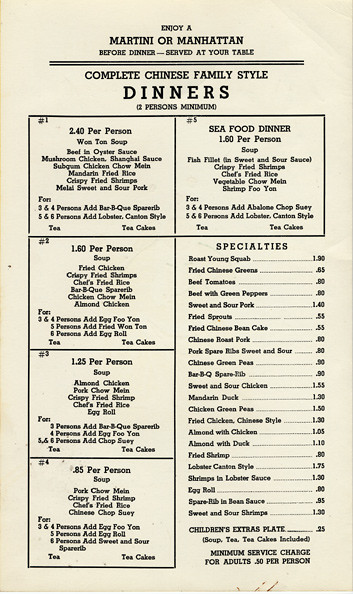In the image, there is a detailed food menu presented against a white background with black text for clarity. At the top of the menu, the text reads "Enjoy a Martini or Manhattan Before Dinner," indicating these drinks are served at your table. Below this, there's another heading that mentions "Complete Chinese Family Style Dinners," with a note that these meals require a minimum of two persons.

The menu is organized into five distinct sections, each within its own square, detailing various food options and associated prices per person:

1. **Square 1**: Priced at 2.4 per person, this section includes Wonton Soup, Beef in Oyster Sauce, Mushroom Chicken, and Spaghetti Sauce.
2. **Square 2**: Priced at 1.6 per person, this section offers a variety of dishes including Soup, Fried Chicken, Crispy Fried Shrimp, Chef's Fried Rice, Barbecue Spinach, and Chicken Chow Mein.
3. **Square 3**: Priced at 1.25 per person, this section features Almond Chicken and Pork Chow Mein.
4. **Square 4**: Priced at 0.85 per person, this section includes Pork Stew, Pork Chow Mein, and Crispy Fried Shrimp.
5. **Square 5**: This is labeled as the Seafood Dinner, priced at 1.6 per person, and it lists all the seafood specials available.

Each section provides a variety of options, offering customers an array of choices to cater to different tastes and preferences. The overall design and layout are clear and visually appealing, making it easy for diners to understand and select their desired meals.